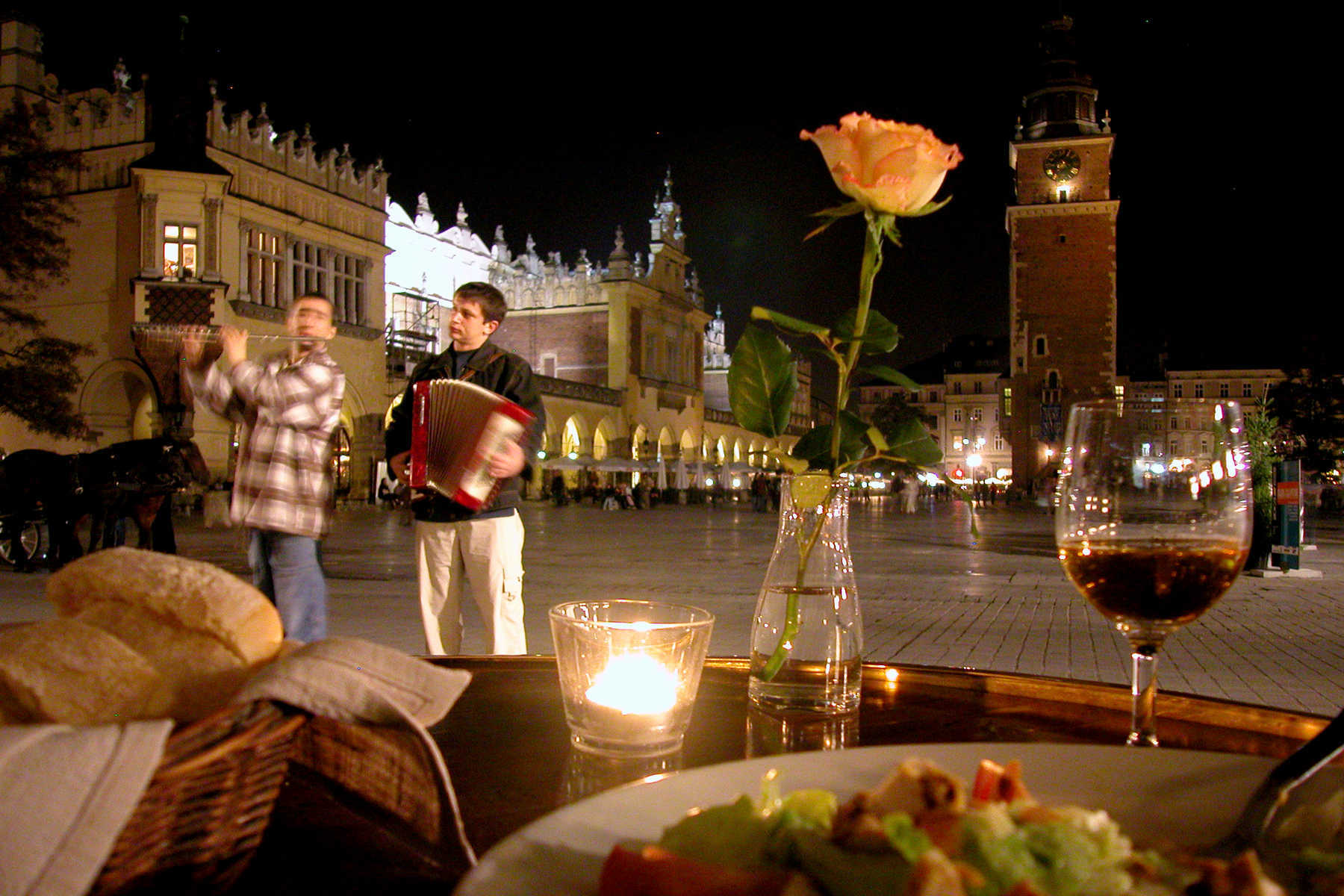In this nighttime scene set in a European city square, a small restaurant table in the foreground holds a lit candle, a pinkish rose in a vase, a glass of wine, and a basket of bread. There's also a white plate with a meal that is partially visible. To the left of the table, two men are performing; one plays an accordion while the other claps or sings. Behind them, a large, illuminated building resembling a castle or clock tower stands out against the dark sky, suggesting a historic or prominent city center, possibly Italian. The area appears to be paved with cobblestones, adding to the charming, old-world atmosphere. The entire scene exudes a picturesque and lively European ambiance, perfect for a tranquil night out.